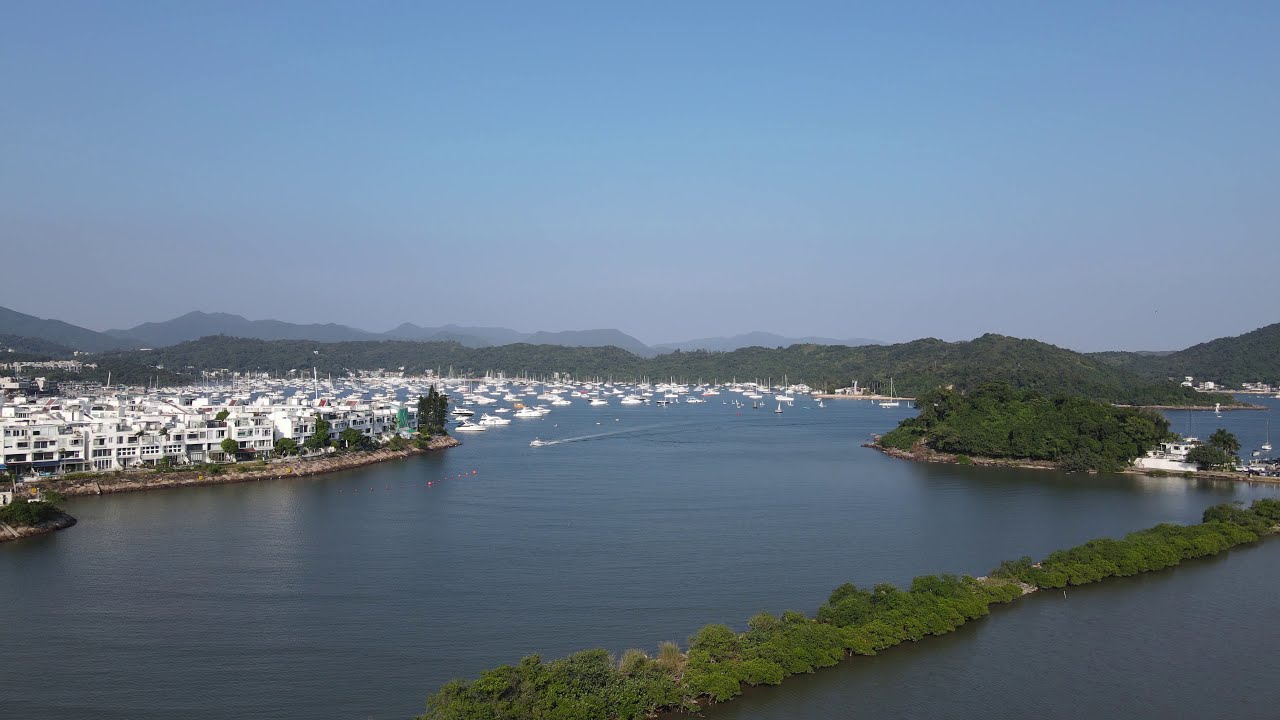The image captures a picturesque view of a serene harbor, showcasing a clear blue sky with no clouds. Set against a backdrop of distant, dense green hills and a darker line of rolling hills, the photograph features a vibrant body of blue-green water at its center. To the left side of the image lies a bustling bay area filled with dozens of stationary white sailboats and yachts, nestled closely within their berths. Just behind this marina, a collection of white buildings and apartment complexes line the natural shoreline. A striking feature in the scene is a stretch of land—an elongated green strip covered in trees—that cuts across the bottom center and extends up to the center right of the image, resembling a small island in the water. Additionally, a small powerboat is captured moving towards the bottom left, leaving a visible wake as it traverses the still waters. The harmonious blend of natural and man-made elements, all framed by the lush green hills, paints a vivid and inviting coastal landscape.